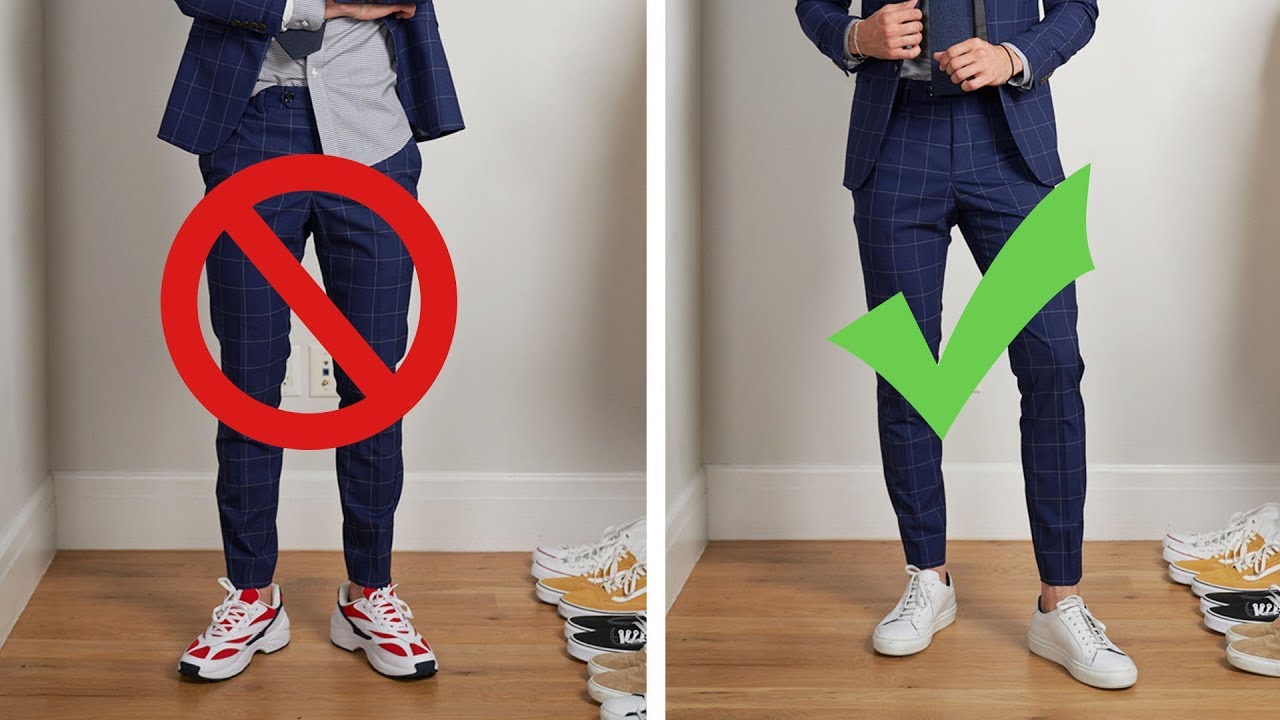The image is a horizontally oriented, two-pane photograph showcasing a 'do and don't' fashion comparison of a young man. The left pane features the man from just above the waist down, dressed in a blue suit with white cross lines forming squares, a light blue shirt untucked, and red and white sneakers. His outfit appears disheveled. The background includes a wooden floor, gray walls with white baseboard, and a visible line of shoes. Overlaying this pane is a red circle with a slash, indicating a 'don't.' In contrast, the right pane shows the same man, but his shirt is neatly tucked in, and he is wearing white sneakers. His attire is polished, with a snugly fitting jacket and visible sleeves, making him look prepared and put together. The background remains unchanged, but a large green check mark overlays this pane, signifying a 'do.'